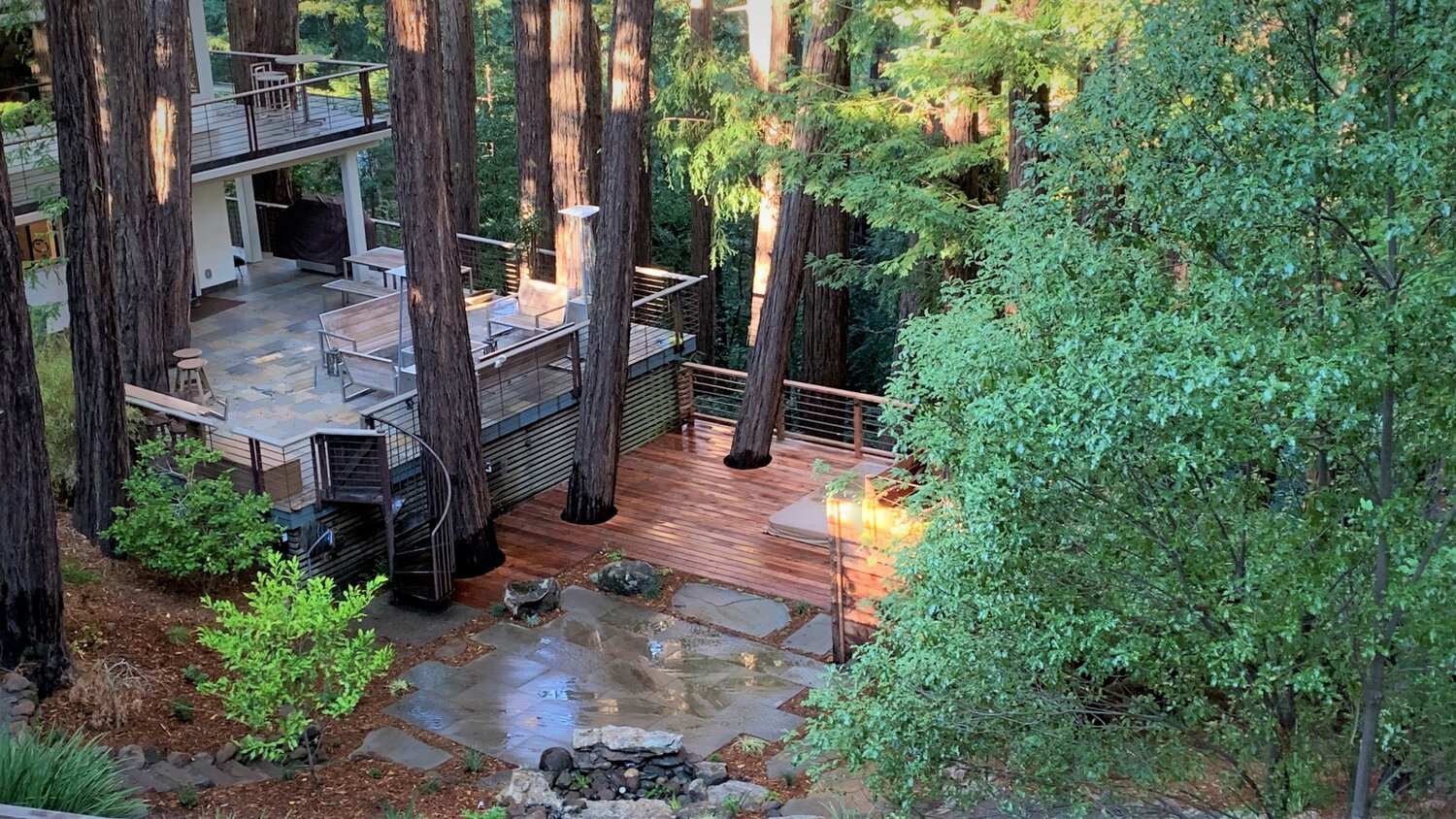This photograph captures a picturesque scene of a forested hillside with a multi-level house seamlessly integrated into its lush surroundings. The house, situated on the left side of the image, features three distinct levels. The lower level comprises a wooden deck with a possible hot tub marked by a light brown cover in the corner, alongside a stone fire pit and a small stone patio. Trees with green, leafy canopies pierce through the deck, indicative of holes made to accommodate them, emphasizing the house’s harmonious design with nature.

Moving upwards, the second level reveals another patio with benches and seating areas enclosed by a dark wooden rail and accessed via a curved stairway. Sunlight filters through the high branches at the top of the photo, casting a warm glow on the scene, highlighting the dark finish of the wood. The highest level boasts an additional balcony supported by visible beams.

The house's exterior is painted white or cream, blending demurely with the verdant environment. A dense array of trees, including a prominent green bush on the bottom left, frames the setting, while the sunlight dapples the greenery, suggesting it is daytime. A grove of tall, thick trees stretches from the middle to the right side, sloping downwards, which complements the hilly terrain on which the house is built. The overall ambiance suggests a serene residence nestled in a thriving forest, bathed in natural light with a slight indication of recent rain as the deck looks wet.